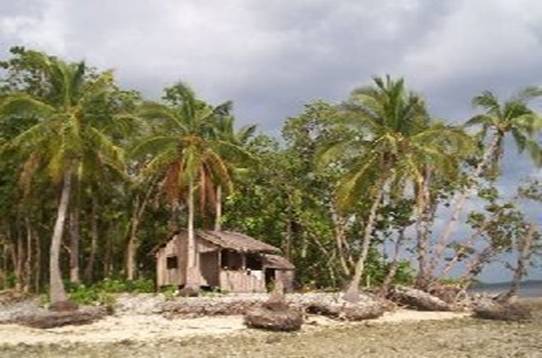This photograph depicts an island scene dominated by a small, tan wooden shack nestled amidst a dense gathering of coconut palm trees and lush greenery. The shack, appearing somewhat aged, suggests that the photograph itself might be older, given its slightly pixelated quality. The shack, possibly consisting of about three rooms, is accompanied by what seems to be a wooden shed to its side. The setting is further enriched by a sandy beach-like area, punctuated with rocks in the foreground. To the far right, one can discern a body of water, likely the sea or ocean. The skies overhead are a mix of blue and gray, with darker clouds indicating the wind blowing, causing the leaves of the palm trees to sway. The overall color palette of the photograph includes shades of gray, tan, green, brown, and of course, the blue of the partial sky.